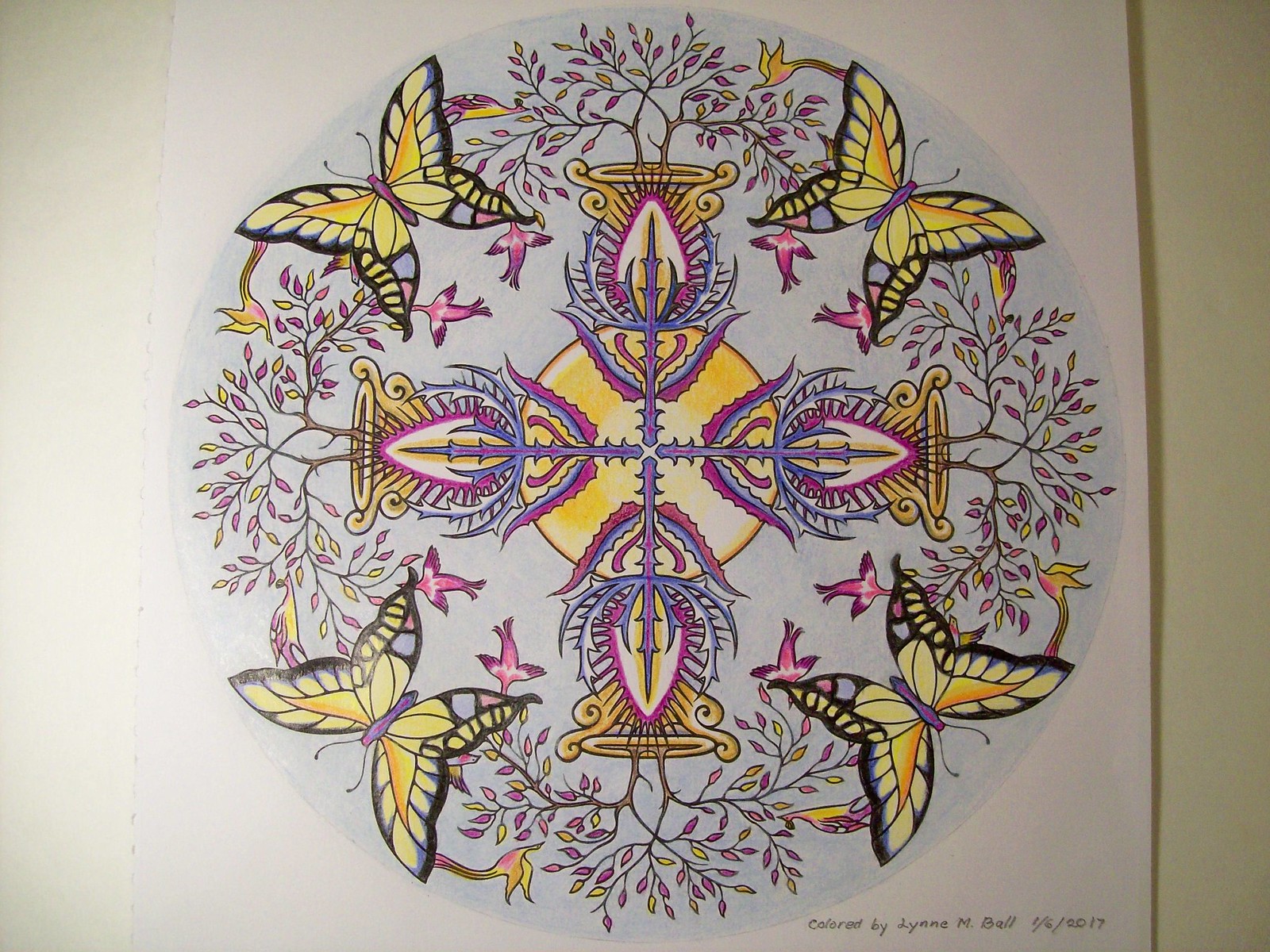The illustration features a central blue circle adorned with intricate patterns, situated on a white sheet of paper. Surrounding this blue circle are four golden pots positioned at the top, bottom, left, and right. These pots are interconnected by a secondary orange circle, which is further intertwined with blue and purple vines.

Each golden pot hosts a tree, each adorned with multicolored leaves including shades of yellow and purple. Between these pots and trees, four butterflies grace the scene, one in each corner. These butterflies sport purple bodies and yellow wings accentuated with blue and purple hues. Additionally, at the base of the wings of each butterfly, there are small pink birds, adding an extra layer of detail to the composition.